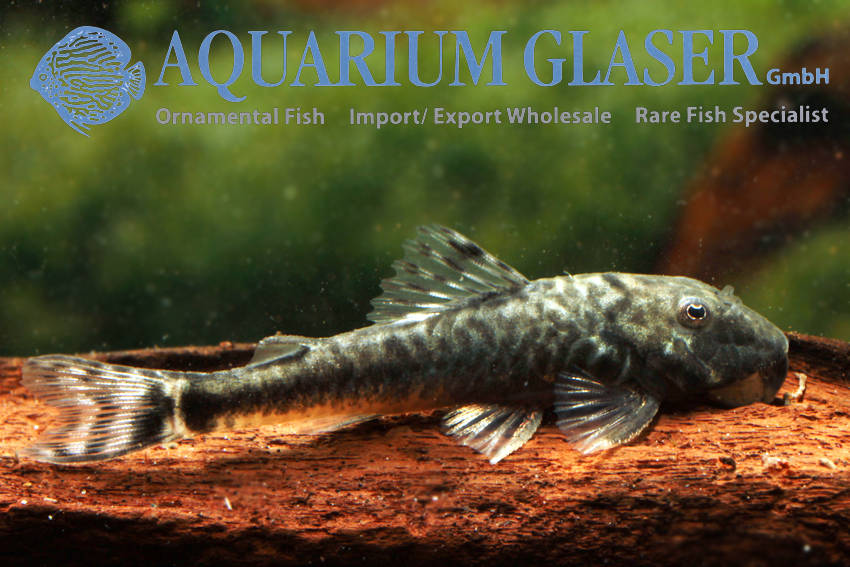This horizontally aligned rectangular image appears to be part of an advertisement or promotional material for 'Aquarium Glacier GmbH,' a company specializing in ornamental fish, import/export wholesale, and rare fish specialists. The upper-left corner features a blue-outlined fish facing left. The company name, "Aquarium Glacier," is prominently displayed in bold blue all caps, followed by "GmbH" in smaller capital letters to the right. Beneath this, gray text reads "Ornamental Fish, Import/Export Wholesale," and "Rare Fish Specialist." 

The background of the image is blurred with shades of green and small water spots, suggestive of an aquatic environment. A piece of wood crosses horizontally in the middle-ground. In the foreground, a distinct fish swims facing the right. It is predominantly gray and white with intricate zigzag lines and shiny silver fins speckled with black spots. The fish's large eye is prominently visible on the right side of its head.